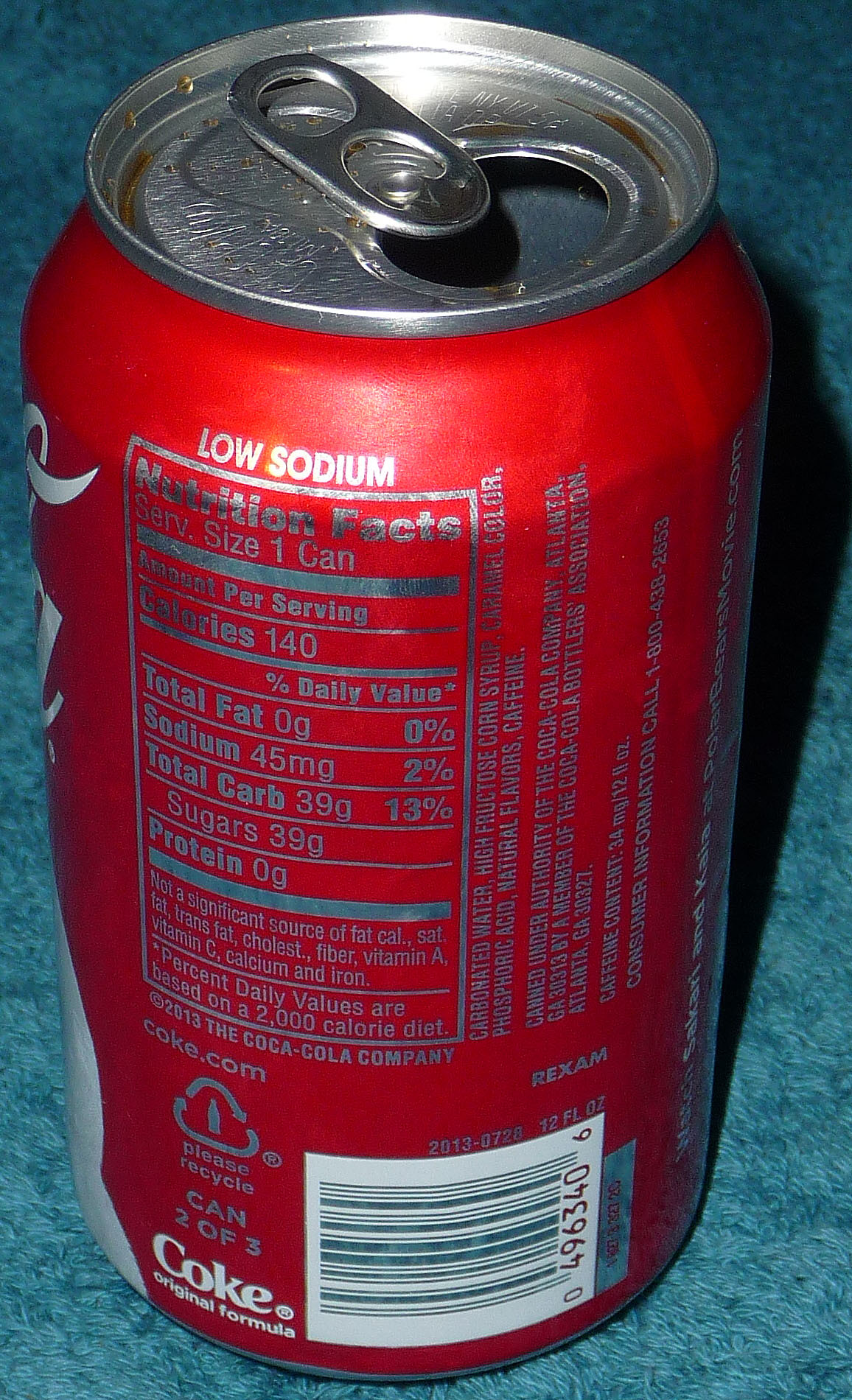This detailed photograph captures the rear view of an open Coca-Cola can seated on a teal-colored surface, likely a blanket or rug, indicated by the visible fibers. The iconic red can, with its nutrition facts label in silver, stands out against the cool backdrop. The can, which is partially consumed, shows remnants of the beverage in the ridge around its opening and droplets of soda. The label includes details about serving size and mentions "low sodium," among other nutritional information.